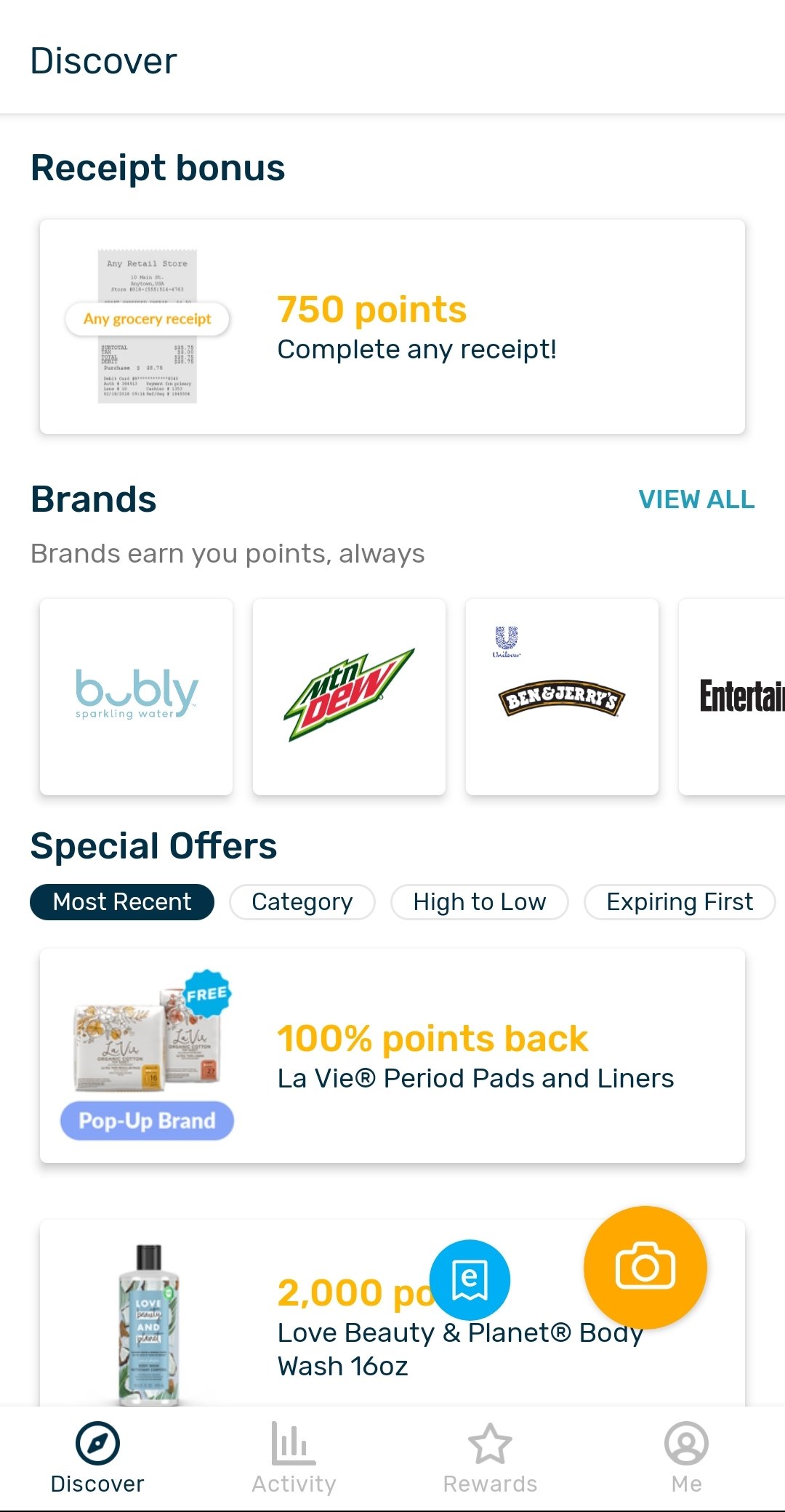This screenshot showcases a promotional app interface. At the top, a navigation tab labeled "Discover" is highlighted, indicating the current section being viewed. Below, there's a featured promotion titled "Receipt Bonus," displayed within a rectangular frame. It reads, "Any grocery receipt," accompanied by an icon of a grocery receipt, and offers "750 points" for submitting any grocery receipt.

Further down, a section labeled "Brands" with a prompt to "View All" is visible. This section highlights the opportunity to earn points from various brands, displaying logos for BUBLY, Mountain Dew, Ben & Jerry's, and another brand partially visible with the text "Entertainment."

Underneath, the "Special Offers" section categorizes deals by "Most Recent," which is currently selected, along with options for "Category," "High to Low," and "Expiring First." Within this section, two promotional boxes are prominently featured:

1. The top box offers "100% points back" for "Free L.A.V.A. Period Pads and Liners," alongside an illustrative product image.
2. The bottom box showcases a "Love Beauty and Planet Body Wash, 16 oz" with an offer of "2,000 points," accompanied by another product image.

At the bottom of the interface, there's a dashboard menu featuring options: "Discover," "Activity," "Rewards," and "Me," providing quick access to various aspects of the app.